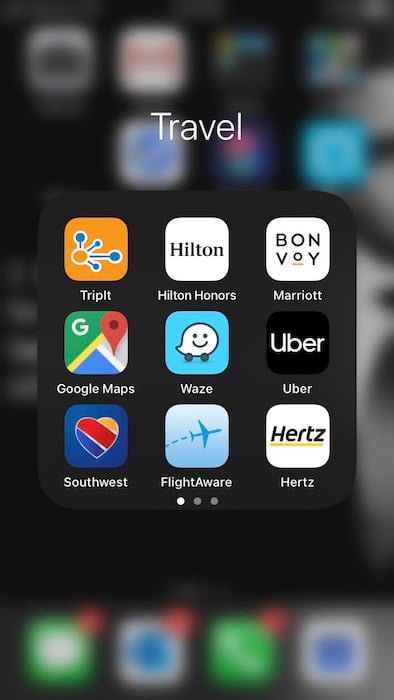A detailed and cleaned-up caption for the image could be:

"This screenshot, captured from an iOS device, prominently features a dedicated travel folder containing various travel-related apps. In the foreground, the 'Travel' folder displays several apps including TripIt, whose icon is orange with blue and orange circles; Hilton Honors, shown with a simplistic 'Hilton' text on a white background; and Marriott, with an icon showcasing 'BONVOY,' where 'B-O-N' and 'V-N-Y' are in capital letters while 'O' is lowercase with a red underline. Also visible are popular apps like Google Maps, Southwest Airlines, and Uber. The background of the image is blurred, bringing the travel apps into sharp focus, with some obscured notifications appearing at the bottom."